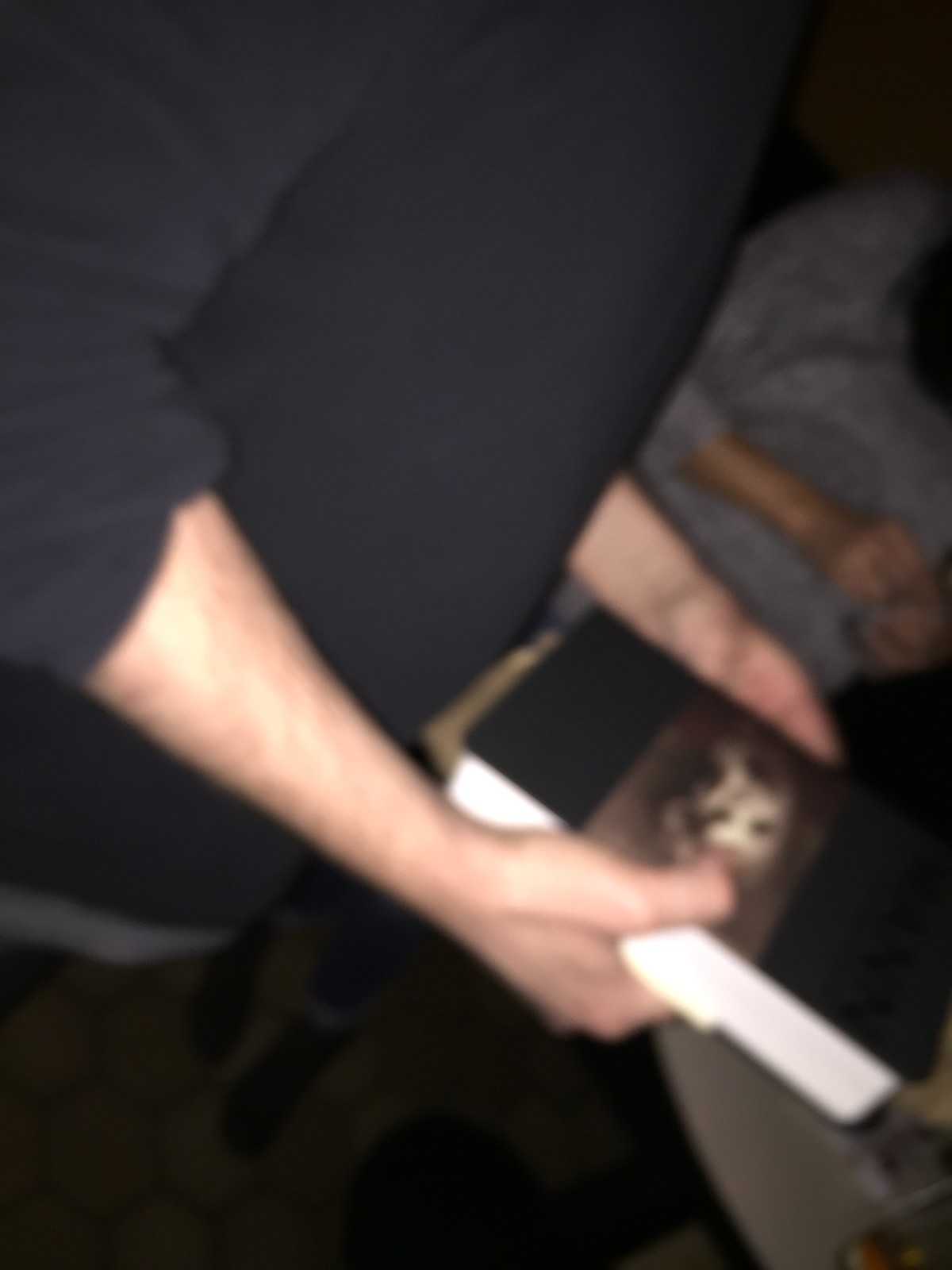The image is a vertically oriented, slightly rectangular photograph taken from a lower left to upper right angle. The scene is dimly lit, creating a dark, moody atmosphere. On the left side of the frame, we see the profile view of a person’s chest and part of their right arm extending down towards the right side of the image. The person's left arm, visible from just below the wrist, extends downwards from the abdomen area. They are holding a book with a black cover, characterized by a horizontal band across the center. This band, appearing in a blurry brown hue, contains an indistinguishable figure, contributing to the mysterious, subdued composition of the photograph.